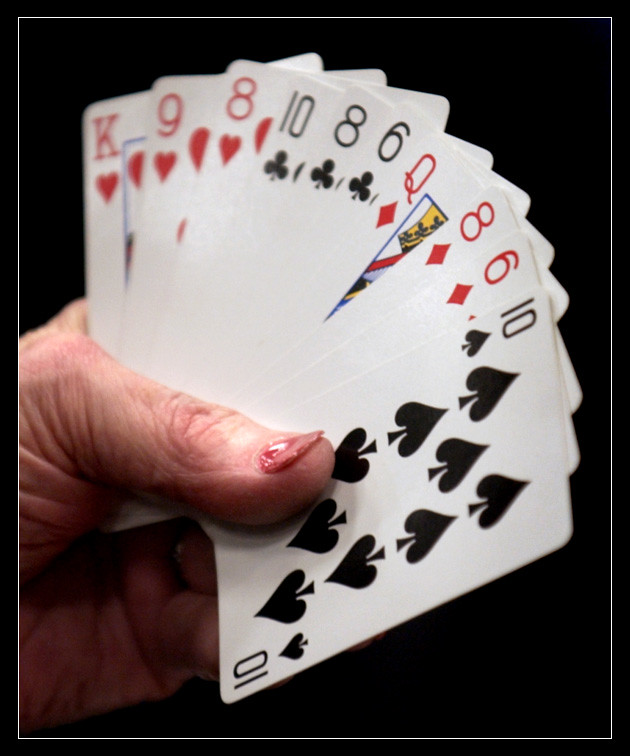In this vivid color photograph, a hand is prominently displayed, holding a fanned out arrangement of ten playing cards, suggesting a card game in progress. The thumb and the heel of the hand are visible on the left side of the image, entering the frame from the left. The thumb nail, which has a slightly spatulate appearance and seems to lift from the flesh of the thumb, is painted in a rather unappealing shade of dark pink-red.

The cards in the hand are as follows: a king of hearts and a queen of diamonds as face cards; three eights; two sixes; a nine of hearts; a ten of spades; and a ten of clubs. The hand, whether dealt or chosen, seems to hold a strong position in the game, though the specific game played remains uncertain. The cards are carefully arranged, with the ten of spades being the most prominently displayed at the far end of the fan. The image is set against a stark black background, offering no additional context or distractions.